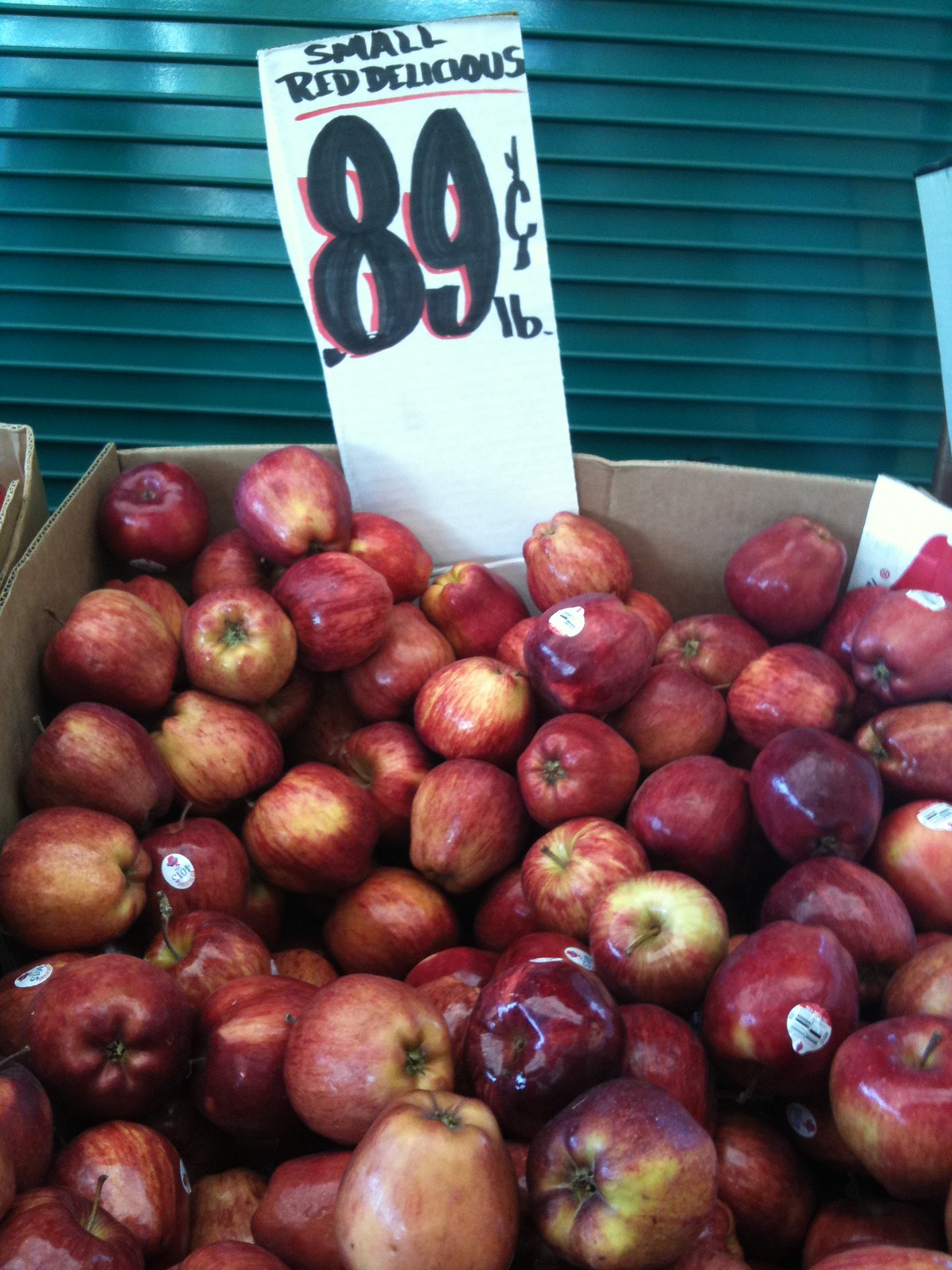This color photograph captures a large, overflowing cardboard box brimming with over a hundred shiny apples. The apples are predominantly dark red, with some exhibiting a mix of red and yellow hues. Each apple has a sticker on it. A handcrafted sign made from white cardboard sits at the back of the box, displaying "SMALL RED DELICIOUS" in bold, underlined letters written in red Sharpie, with the price listed as "0.89¢ LB" in large handwritten numerals. The box is positioned against a teal-colored industrial metal wall, similar to a roll-down garage door, adding a distinct backdrop. To the left and right of the main box, edges of other cardboard boxes are faintly visible. This image likely serves to advertise the apples and their price.